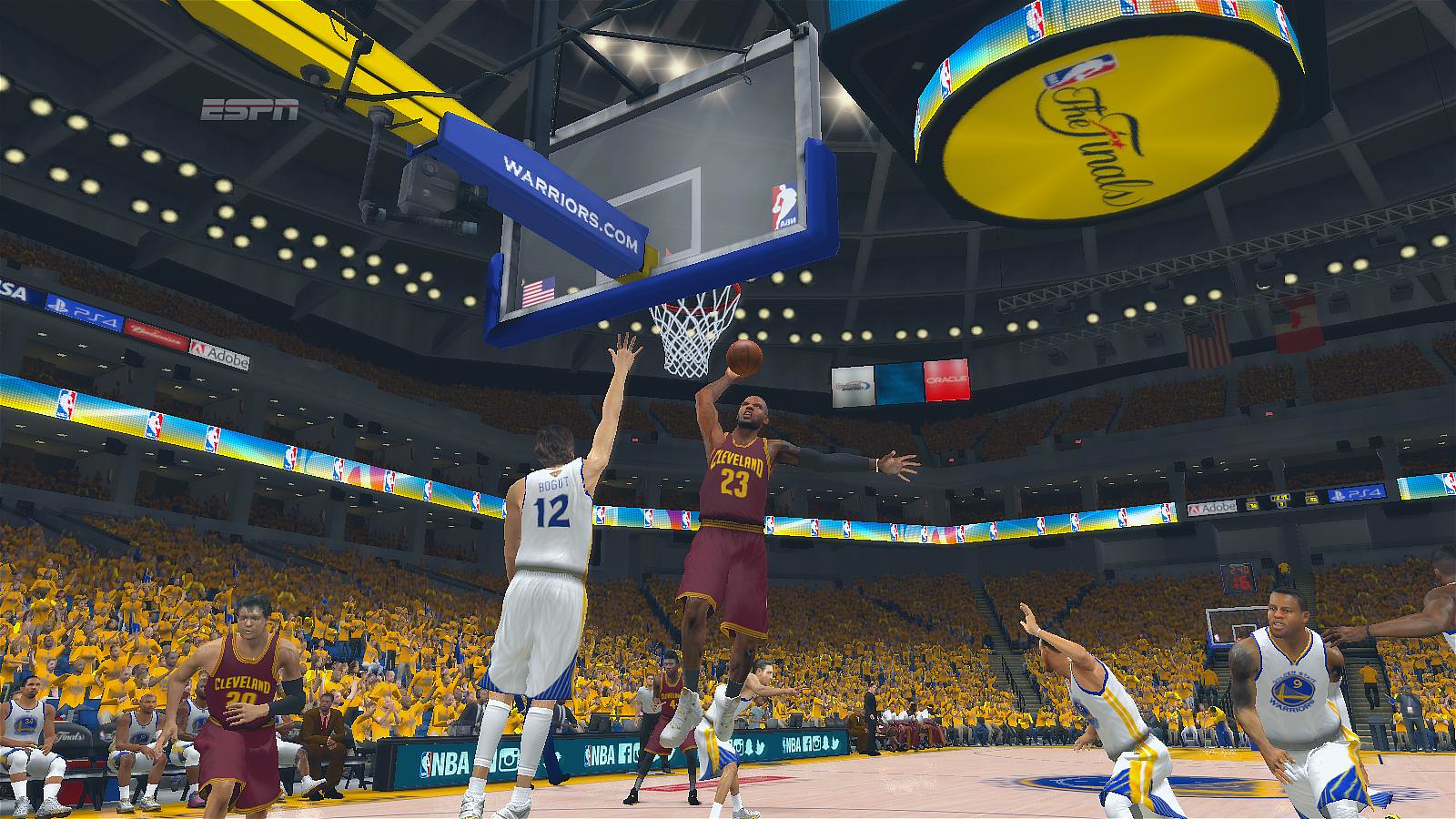This highly detailed computer rendering, most likely from the NBA 2K video game series, captures an intense moment in a virtual NBA Finals recreation. In this scene, set in a packed stadium immersed in the vibrant atmosphere of a Golden State Warriors home game, two teams face off in a dynamic basketball play. The court, comprised of light-colored wood, features prominently visible graphics, including the NBA logo and "The Finals" branding, both of which are captured on the floor. The focal point of the image is two players mid-air: a darker-skinned player from the Cleveland Cavaliers, wearing a burgundy and gold jersey, appears to be executing a powerful dunk while his lighter-skinned opponent from the Golden State Warriors, dressed in a white, blue, and gold uniform, attempts to block the shot. The background immerses viewers in the virtual crowd, most of whom are adorned in Warriors' yellow shirts, underscoring the home court advantage. The realism extends to the court details with visible elements like the ESPN watermark in the top left corner and the Warriors.com branding on the basket stanchion, further enhancing the authentic feel of the video game imagery.